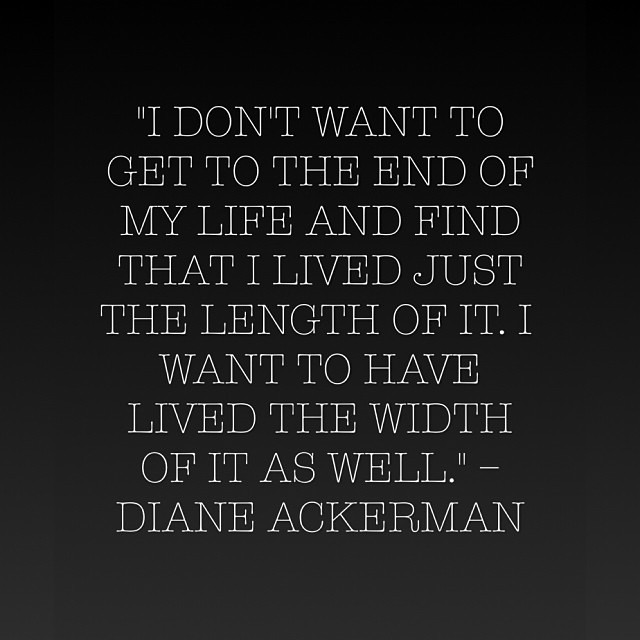The image is a black and white graphic featuring a powerful quote by Diane Ackerman. The background is predominantly black, with a subtle gradient shading to a very dark grey towards the bottom, enhancing the stark contrast with the white text. The text itself is in a distinctive serif typewriter font, with unique characteristics such as horizontal lines on the tops of T's, L's, W's, and A's, which adds a vintage charm. The quote reads: "I don't want to get to the end of my life and find that I lived just the length of it. I want to have lived the width of it as well." Diane Ackerman's name is clearly attributed below the quote. The image is minimalistic, fully focused on the message, with no other elements or images present, highlighting the motivational and introspective essence of the quote.